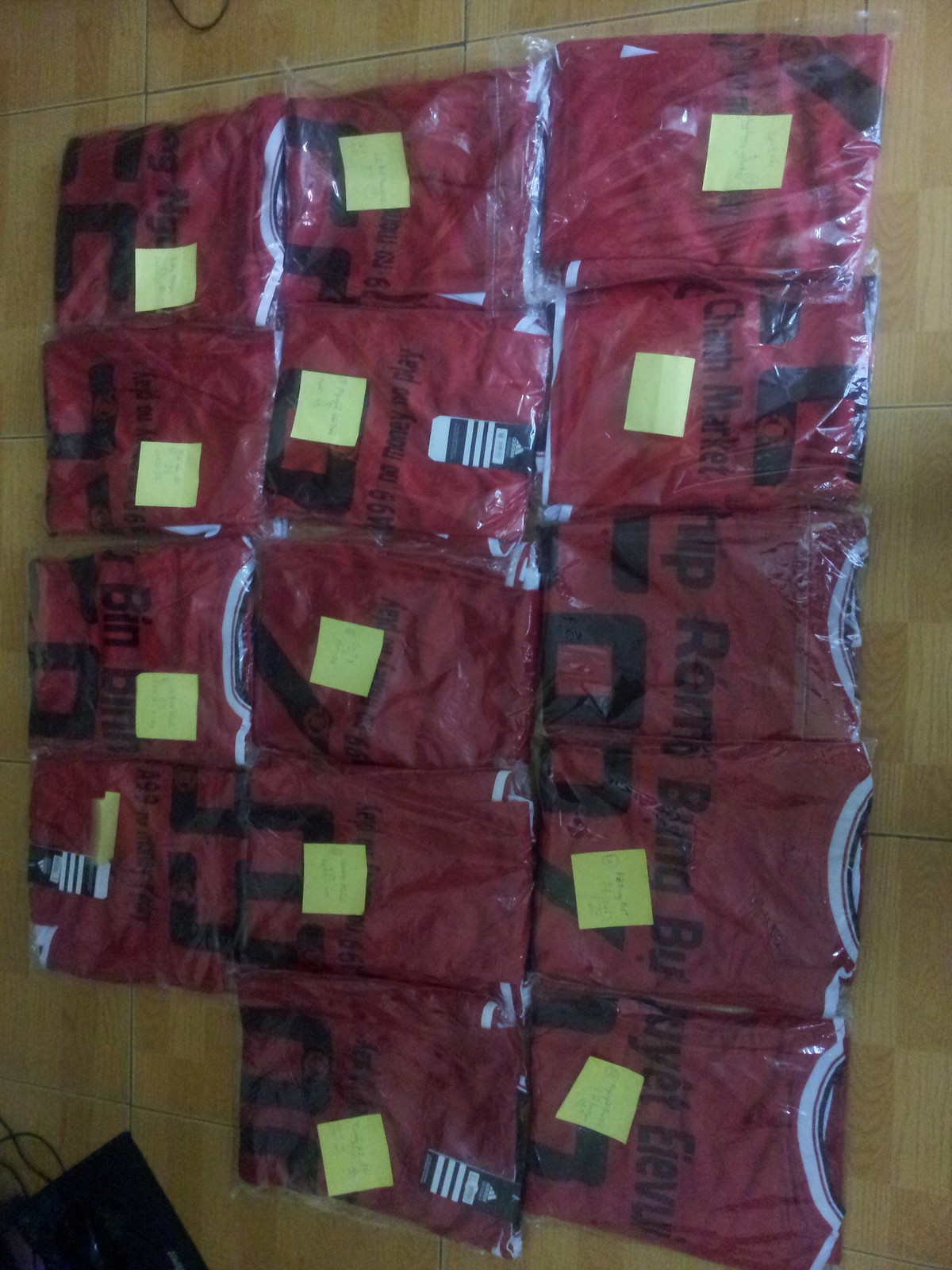This image is a vertical rectangle shape, likely turned 90 degrees counterclockwise from its original horizontal orientation. The background appears to be a hardwood floor, or possibly fake wood floor tiles, featuring a subtle checkerboard pattern of light and dark brown hues. Arranged on the floor are 14 plastic-wrapped packages, each containing what seem to be red uniforms, possibly jerseys or t-shirts. These packages are neatly organized in rows: four on the left, five in the middle, and five on the right. Each uniform bears black text, likely names and numbers, though the text is in a foreign language and partially obscured. Additionally, almost all packages have yellow sticky notes affixed to them, the content of which is unreadable.